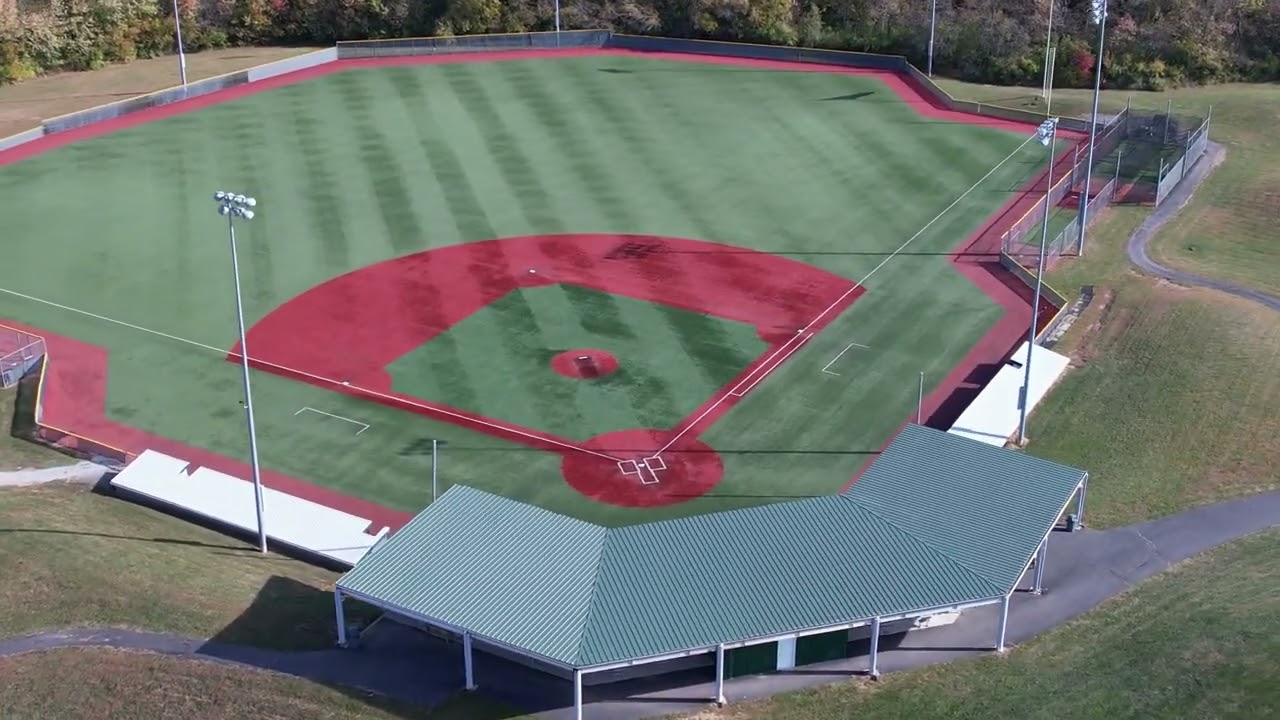The image captures a beautifully manicured, empty baseball field, likely belonging to a high school due to the absence of extensive stands. The field features a reddish earth baseball diamond and an outfield warning track that frames the playing area, giving it a distinct, polished look. The varying shades of the freshly mowed grass form a pattern of dark and light green stripes, highlighting meticulous care. The entrance to the field is marked by a green slatted roof supported by white metal poles, with dugouts on either side having white roofs. Large lights are strategically placed around the field, indicating it accommodates night games. Surrounding the field is a grassy expanse, with a pathway visible to the right and more grass to the left. In the distance, a backdrop of numerous trees adds a serene, natural setting to this tranquil sporting venue.